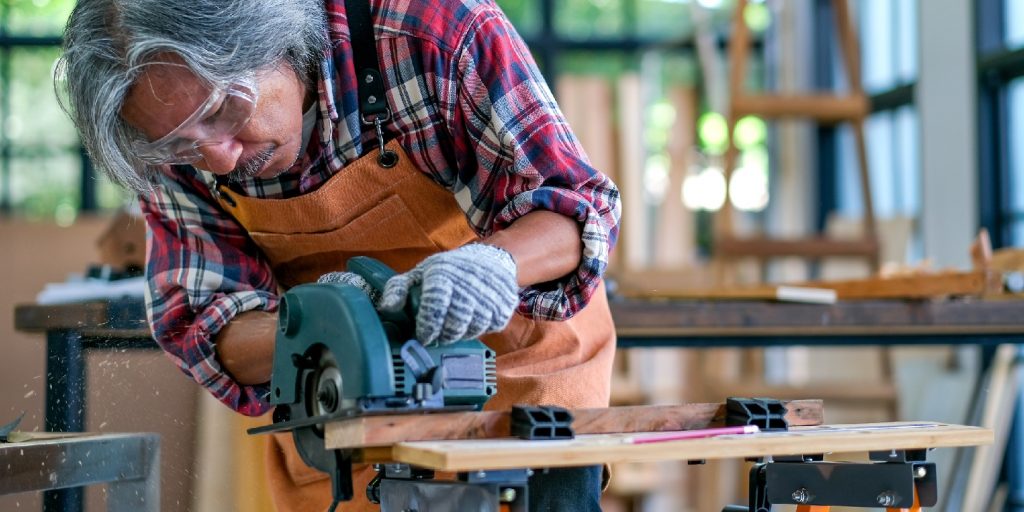The image showcases a meticulous woodworker in his garage workshop, engaged in the precise task of cutting a 2x4 piece of lumber with a blue hand saw. He is protected with clear safety goggles and blue-and-white gloves, underscoring his commitment to safety. The woodworker, an older man with gray hair and a gray beard, wears a checkered shirt and overalls. His intense focus is evident as he measures and cuts the wood, with a pink pencil resting on a piece of wood indicating his precision. Behind him, a broader scene of his workspace reveals a brown table atop which sits an upside-down chair, black-framed windows, and a brown ladder in the corner. The well-lit room shows him deeply immersed in his craft, surrounded by various woodworking tools and materials.